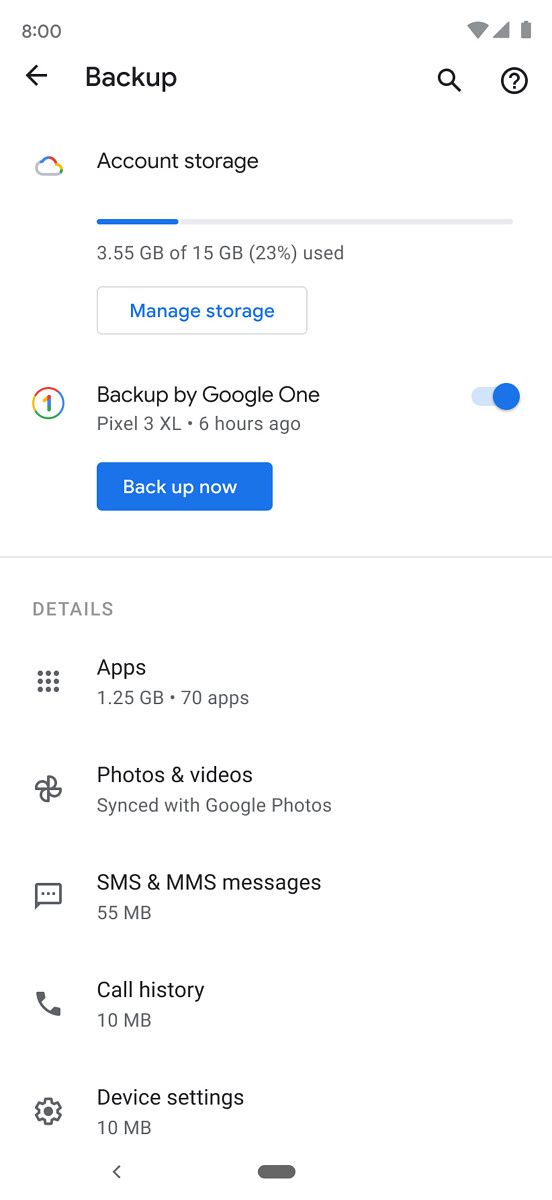**Detailed Caption:**

In the upper left corner of the image, the time is shown in gray text reading "8:00." The network signal, Wi-Fi, service signal, and battery indicators are all depicted as being fully functional.

In the row below, a black arrow points to the left, followed by the word "Backup" in bold black lettering with a capital "B." On the right-hand side of this row, there is a black magnifying glass icon, followed by a circular outline with a black question mark inside a white circle.

Further down, there is an illustration of a multi-colored cloud in gray, blue, red, yellow, and green. Next to this cloud, the text "Account Storage" is written in black. Directly underneath, there is a horizontal line with segments in blue and gray. The text "3.55 GB of 15 GB (23% used)" appears in gray.

Below this section, a white rectangle outlined in gray contains blue text that reads "Manage Storage." Another section follows with a numbered circle featuring Google’s colors (red, yellow, green, and blue) and the black text "Backup by Google One." Beneath this is "Pixel 3 XL" in gray, accompanied by a gray circle and the text "6 hours ago" also in gray.

A blue rectangle with white text states "Backup now," followed by a horizontal gray line. Below this line, detailed information is provided in black and gray text:

- Apps: 1.25 GB, 70 apps
- Photos and videos: Synced with Google Photos
- SMS and MMS messages: 55 MB
- Call history: 10 MB
- Device settings: 10 MB

The completion of the image is marked by the end of a rectangular shape extending to the left-hand side.